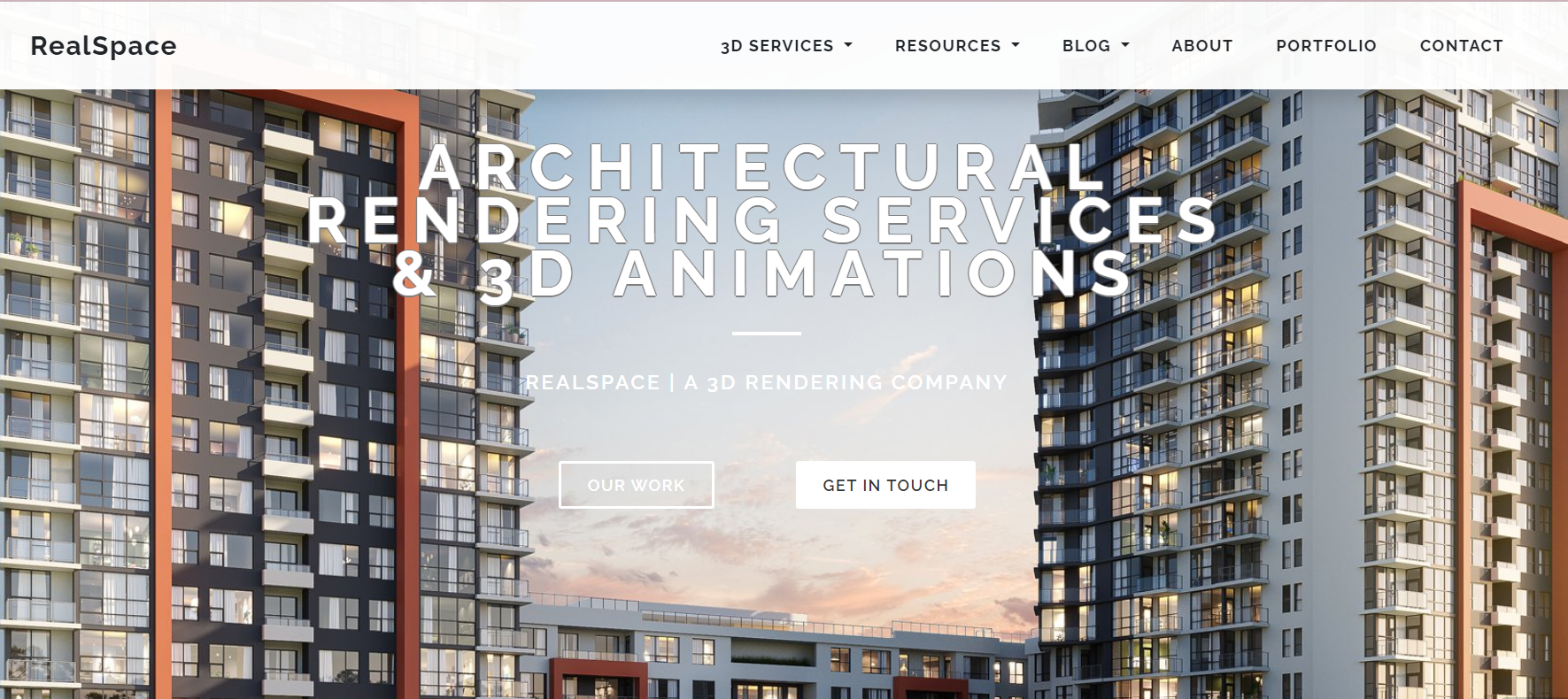This is a cropped screenshot of the desktop webpage for Real Space, a company specializing in architectural rendering services and 3D animations for commercial construction. The background of the webpage features a vivid photo displaying a pair of twin buildings, one on the left and the other on the right, set against a sky that's beautifully hued with shades of blue and pink. At the top, a large white text overlay prominently reads, "Architectural Rendering Services and 3D Animations." Beneath it, in smaller white letters, the text states, "This is Real Space, a 3D rendering company."

Further down, on the left side, there's a white outlined box labeled "Our Work." To the right of it, another white box reads "Get in Touch" in black letters. At the very top of the page is a semi-transparent white header, which allows portions of the background to be faintly visible. The top left of this header displays the bold black text "Real Space." On the right side of the header, there are various category links, including "3D Services," "Resources," "Blog," "About," "Portfolio," and "Contact."